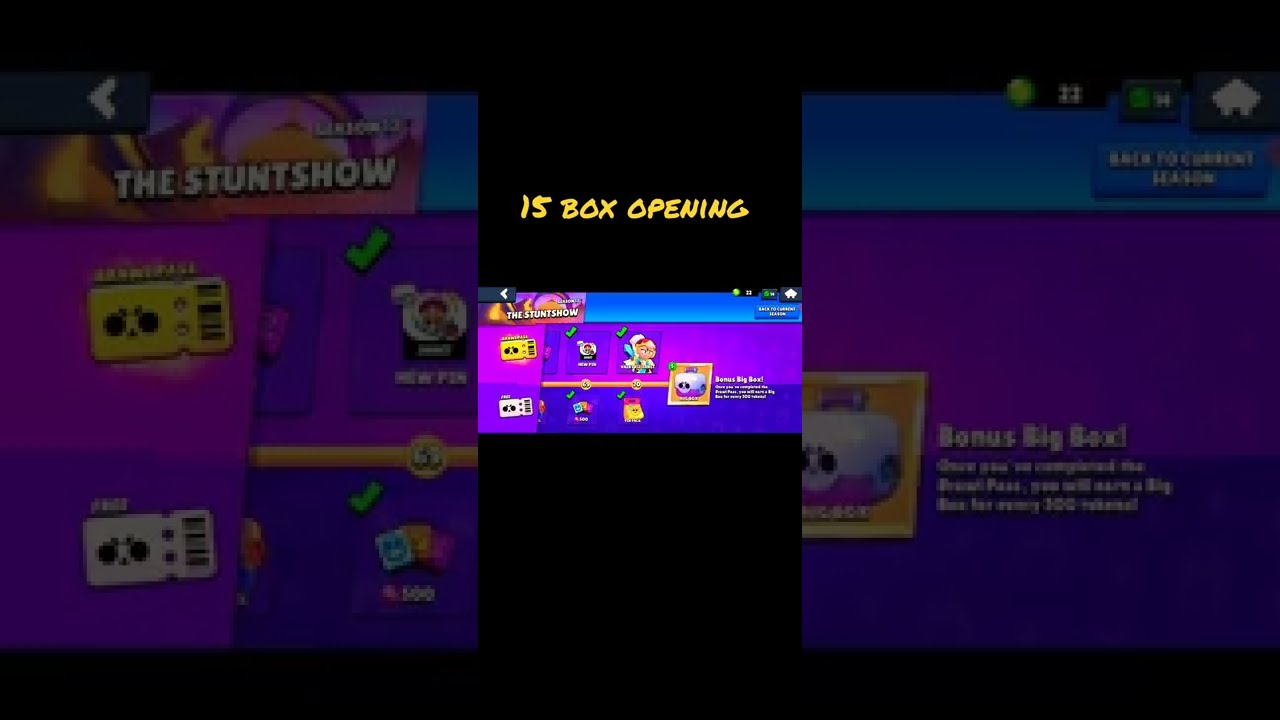This image is a detailed and vibrant screenshot from a video game, specifically from a feature resembling a prize shop or "golden pass" area where players can complete tasks to earn rewards. The main section of the image displays an array of various prizes against a striped backdrop of light and dark purple hues, accented by a blue banner. Prominently, the top left corner of the screenshot features the text "The Stunt Show," indicating a themed event or feature within the game. Centered at the top against a black background, the phrase “15 Box Opening” is written in yellow, handwritten-style capital letters, adding a sense of excitement or anticipation. On the right side, there's a noticeable home icon, suggesting navigation options. Scattered throughout the image are small character icons, tickets, and checkmarks, though many details remain indistinct due to blurriness. The color palette is diverse, including shades of black, white, blue, pink, purple, orange, yellow, green, red, and light blue, contributing to a lively and engaging visual experience indicative of a recreational video game setting. Surrounding this central area are darker, close-up sections of the middle screenshot, giving the entire image a wide rectangular layout.